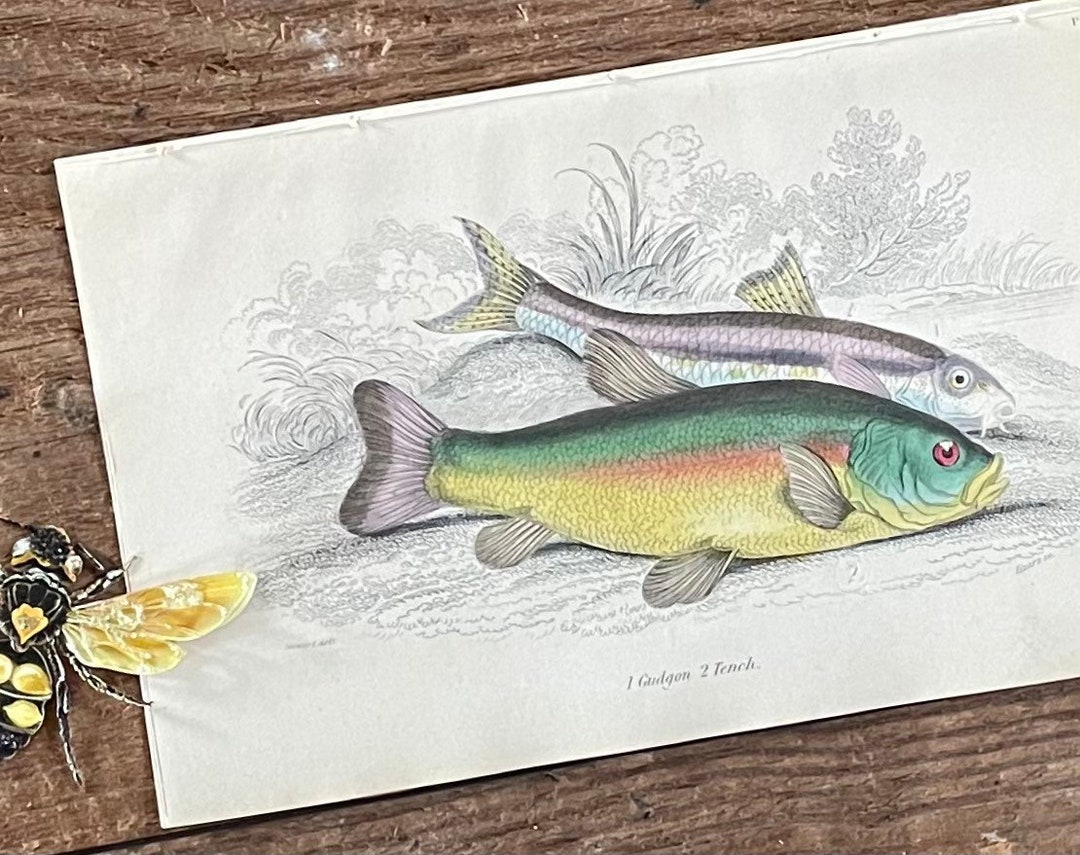The image features an intricate hand-drawn illustration on a piece of paper that showcases two fish against a detailed black-and-white pencil sketch background. The foreground fish, depicted with an emerald green top, a yellow belly, a reddish stripe along its side, and an orange eye, is identified as a "Gudgeon" and is labeled with the number one. The scales on this fish are meticulously detailed, and a fin is prominently displayed. The background fish, reminiscent of a catfish, has grayish-blue hues with silvery accents, whiskers, and fins highlighted with yellow featuring black dots. This fish is labeled as "Tench" with the number two. Both fish are illustrated as if they are resting on a bank near some water, while the surrounding scene includes finely drawn bushes, offering a realistic natural setting. In the bottom left corner of the paper, there is an elaborately colored mud dauber wasp, distinguished by its black body and yellow markings. The entire illustration is laid out at an angle on wooden boards, emphasizing its hand-crafted nature.